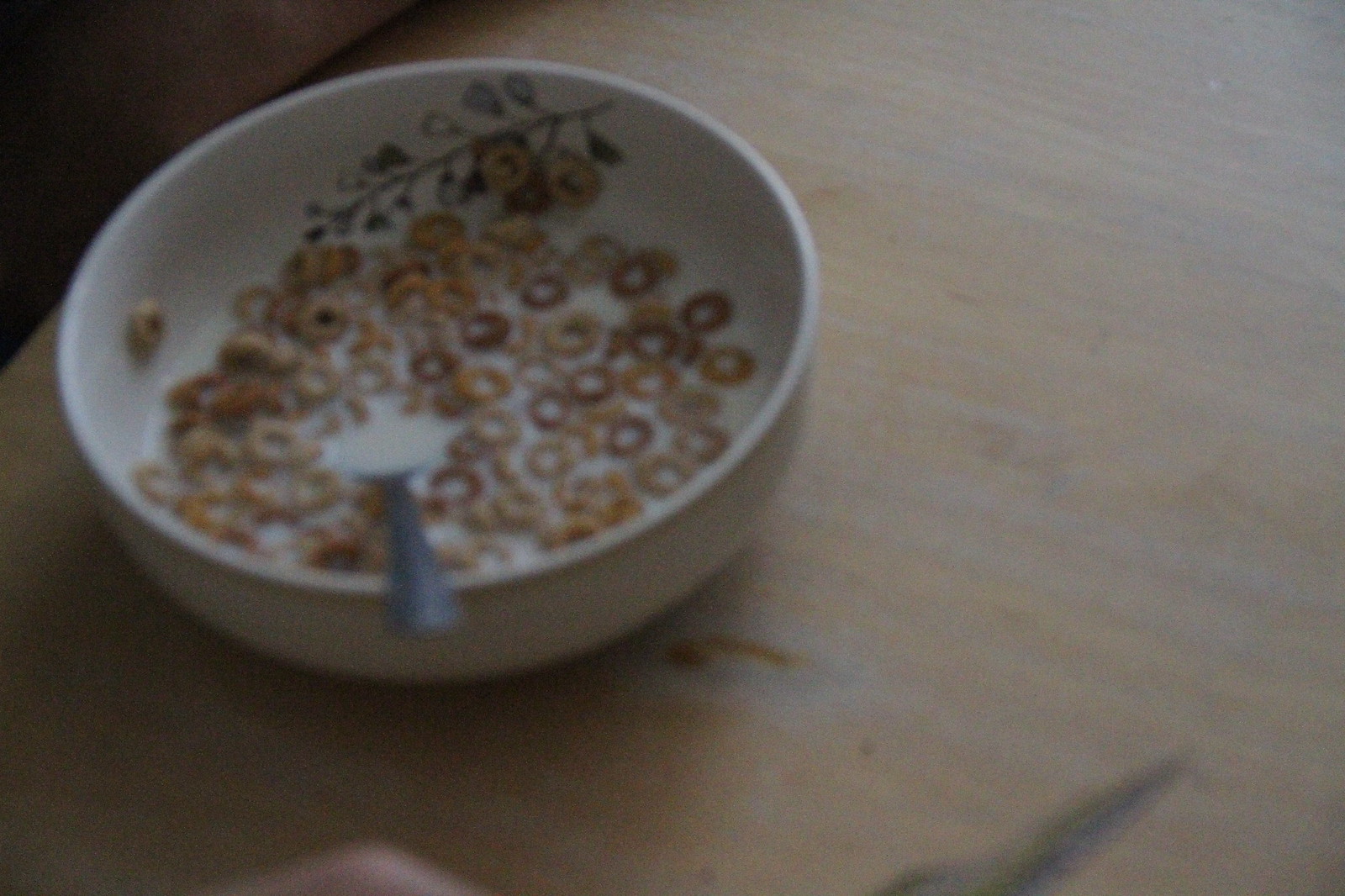The photo, taken in landscape mode, shows a slightly blurred and grainy image of a bowl of cereal. The bowl is filled with O-shaped cereal resembling Cheerios, in various shades of brown and beige, floating in milk. A silver spoon is submerged in the cereal, with its handle resting on the edge of the bowl, protruding towards the camera. The round bowl, which is white and shallow, features a floral and leafy design on its inner rim, consisting of small branches with green leaves and flowers in hues of blue, purple, and white. The bowl is placed on a light brown wooden table. In the blurry background, part of a light-complected finger is visible on the lower left, and there's a black splotch on the lower right side of the image.